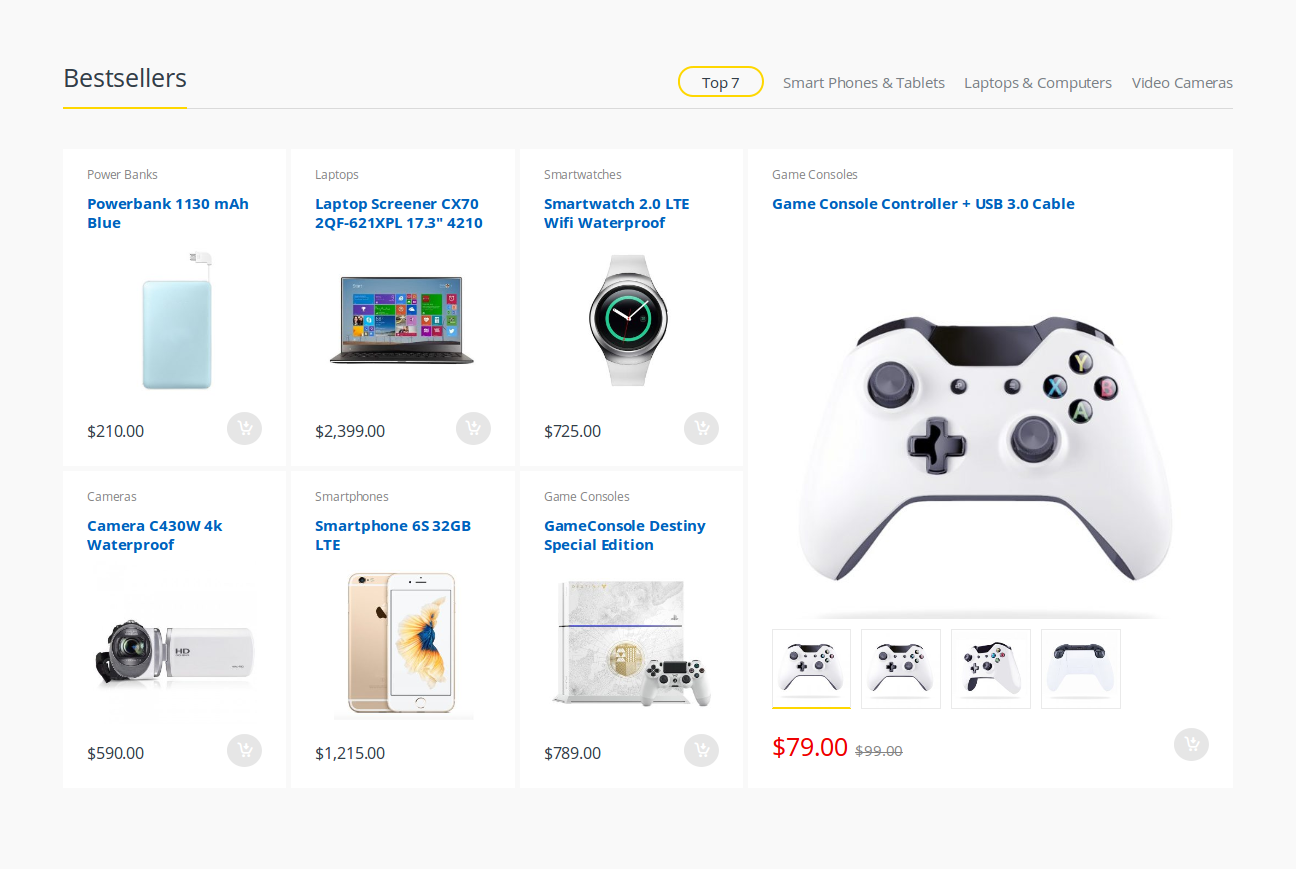The image showcases an electronics shopping website, prominently featuring a range of best-selling products. The top left section is highlighted with the word "Bestsellers" underlined in yellow. Directly below, a horizontal divider spans the width of the page. Encircled in yellow, the phrase "Top Seven" is prominently displayed.

Below the divider, the categories "Smartphone and Tablets," "Laptop and Computers," and "Video Cameras" are listed sequentially. 

The main section of the page displays various product listings:
   
- A power bank with a capacity of 1130mAh, available in blue, priced at $210.
- A 17.3-inch laptop with the model number CX702QF-621XPL, priced at $4210.
- A smartwatch with 2.0 LTE, Wi-Fi capabilities, and waterproof features, priced at $725.
- A game console controller bundled with a USB 3 cable.
- A waterproof camera priced at $590.
- A smartphone model LTE 65, boasting 32GB and LTE capabilities.
- A special edition game console named Destiny. 

Additionally, the website features a rotating view of different game console controllers, showcasing images from the front, back, and side. Various smartphones are listed with prices, one specifically noted at $1,215.